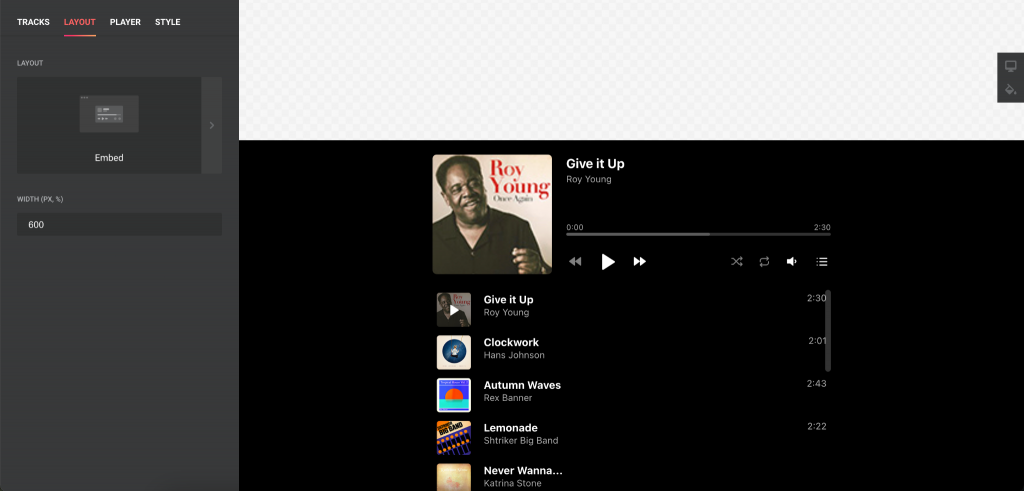The screenshot depicts a user interface for selecting and playing music tracks. The interface is rectangular, approximately six inches wide and three inches tall. On the left side, occupying about one-fifth of the width, there are navigation tabs labeled "Tracks," "Layout," "Player," and "Style." These tabs likely provide different options and settings related to the music and interface customization.

To the right of these tabs, the majority of the screen displays a grayscale background with functional icons, which may represent user account options or additional settings. Below this section, there is a prominent image of Roy Young, an African-American musician, accompanied by the title "Give It Up," suggesting it is the currently selected song.

The interface also lists other song titles, including "Clockwork," "Autumn," "Waves," "Lemonade," "Never," and "Wanna," though it is unclear if they are by the same artist. Functional controls for the music player are also visible, allowing the user to adjust the volume, skip forward or backward, and play or pause tracks, providing a comprehensive, interactive music listening experience.